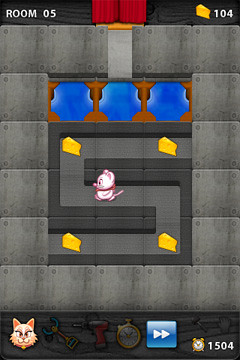The image is a screenshot from a mobile game app featuring a simple, maze-based puzzle. The primary colors used in the interface are gray and blue, with additional splashes of color including yellow for the cheese, brown, and a hint of red. At the very top of the screen, there is a black banner with the text "Room 5" displayed prominently. Below this, there's an illustration resembling a curtain.

In the center of the screen, a small character is seen navigating through a maze. Scattered throughout the maze are pieces of cheese that the character is presumably trying to collect. On the right side of the screen, there is an icon of cheese with a number next to it, indicating "104."

Near the bottom of the screen, the interface features an image of a cat and several blurred-out tools or menu options. The current time is displayed at the bottom right corner. The overall design suggests the game is a casual maze puzzle, intended for light entertainment and to pass the time.